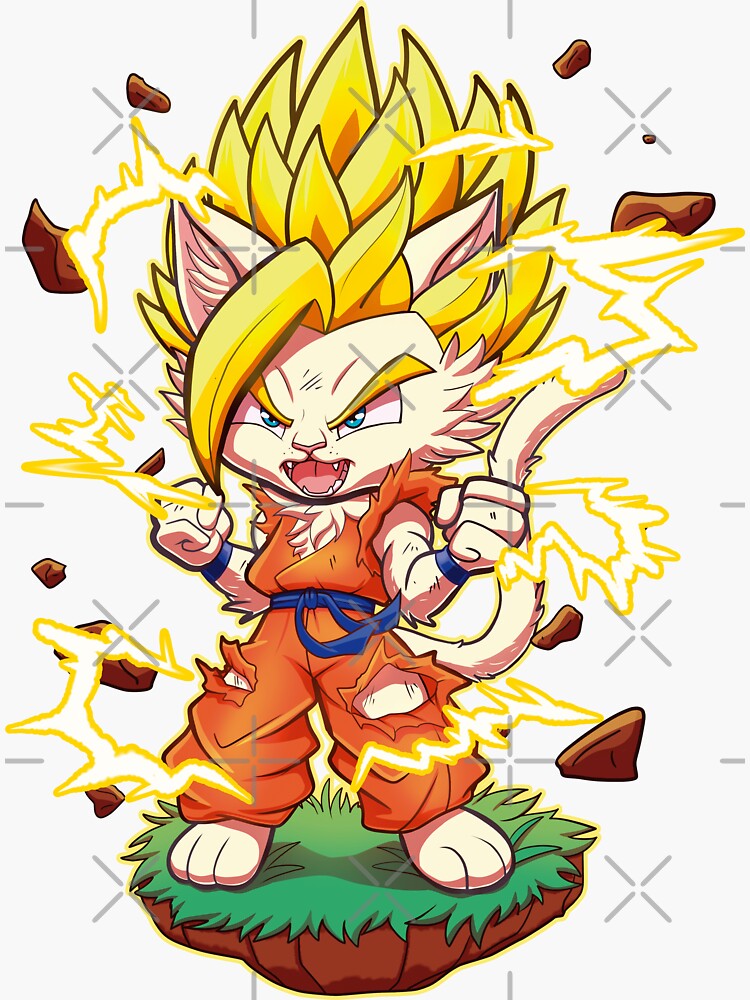The image is a detailed digital illustration of a fierce cat character inspired by Dragon Ball Z. The character, centered in the image, features vibrant pink fur and pointy pink ears. Their hair, spiky and radiant, has turned yellow and is depicted as floating upward, resembling flames, with yellow electricity sparking around it, contributing to a powerful, otherworldly aura. 

This cat is adorned in a tattered orange martial arts jumpsuit, ripped at the knees, with a blue belt knotted at the waist and matching blue sashes around its wrists. The cat’s stance is dynamic, with fists clenched and extended forward, displaying a menacing snarl that reveals sharp fangs, indicating it's ready for battle. The character appears to be standing atop a circular, floating rock platform covered in green grass, with the underlying dirt visible. Surrounding the rock platform and the cat, small brown rocks are suspended in midair, enhancing the dramatic intensity of the scene. The background is stark white, intersected by a few crossed lines, keeping the focus on the electrifying and intense cat warrior.